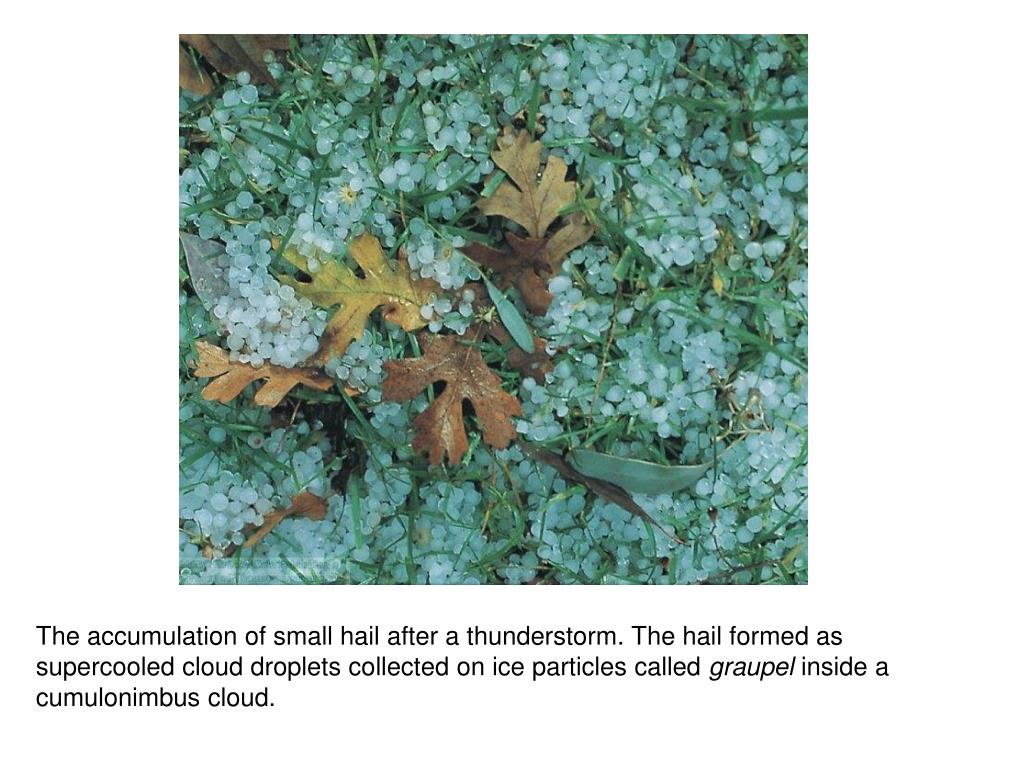A close-up photograph captures the aftermath of a thunderstorm, showcasing the accumulation of small hailstones—formed from supercooled cloud droplets collecting on ice particles known as graupel—scattered across the ground. The hailstones, which are light blue in color and a few millimeters in size, cover the outdoor surface extensively. Amidst the hail, clusters of green grass sprouts break through, and brown leaves are dispersed across the scene, with some leaves centrally placed and others located towards the left and the upper left corner. The image, which has a square dimension, features text in black lettering beneath it: "The accumulation of small hail after a thunderstorm. Hail formed as supercooled cloud droplets collected on ice particles called graupel inside a cumulonimbus cloud." The word "graupel" is italicized to emphasize its definition. The colors present in the photograph include shades of brown, green, turquoise, yellow, and black.